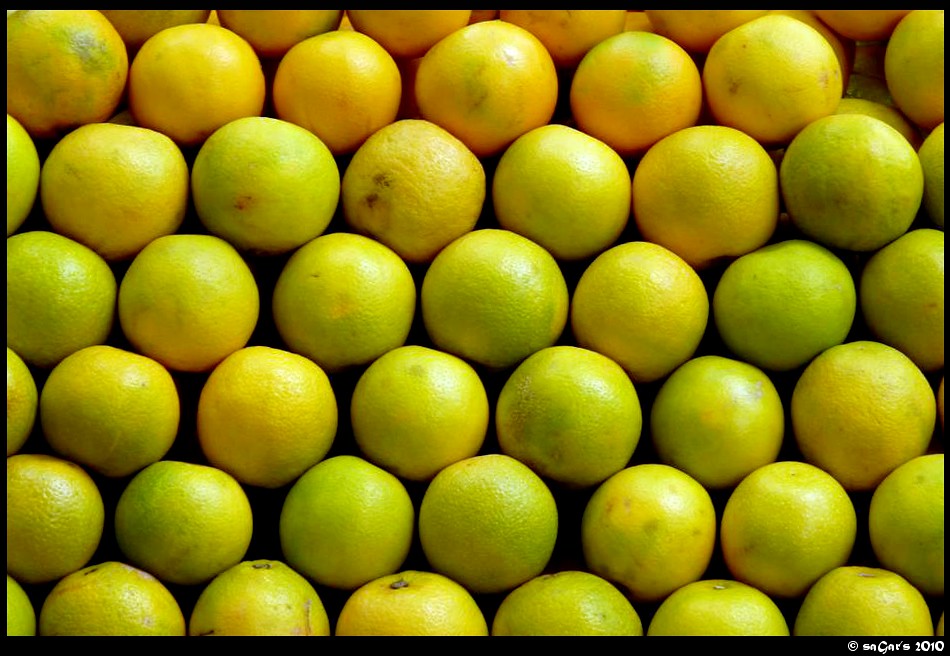This is a close-up photograph of stacked citrus fruits taken from an upper view, capturing a variety of colors and ripeness stages. The fruits, predominantly lemons, are tightly packed together, covering the entire frame in rows. They exhibit a diverse palette ranging from bright yellow to orange, with some greenish hues suggesting a mix of maturity levels. The upper rows feature mostly ripened fruits, while the lower rows hold greener ones. The rind textures vary, with some showing minor imperfections such as small brown spots. The photograph is bordered in black on the lower right corner, where white text, likely the artist's name, and the year 2010 are inscribed, indicating this is a professional and well-composed shot. Overall, the arrangement and lighting create subtle shadows between the fruits, enhancing the visual depth of what appears to be a display of citrus fruits in a produce section.